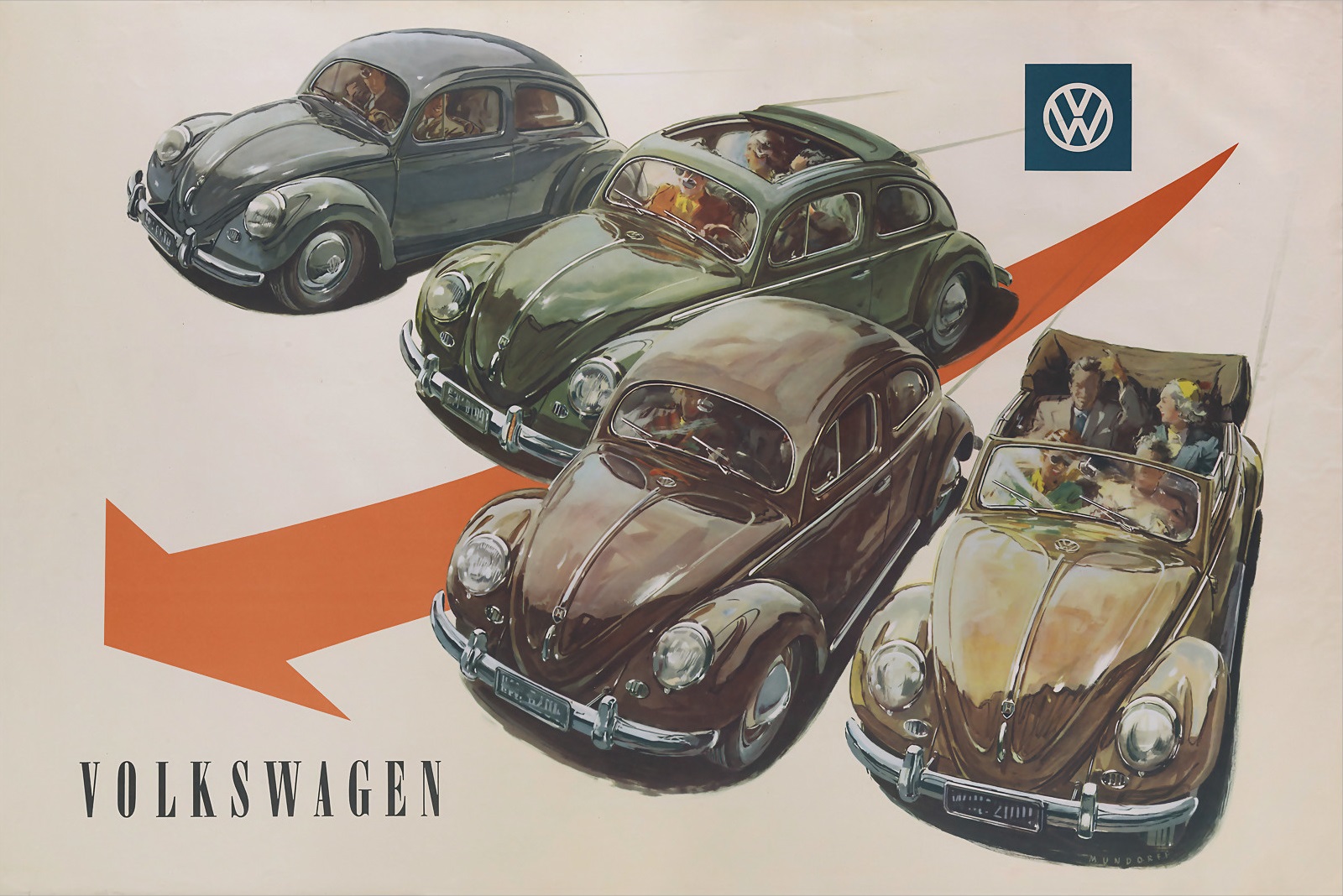This vintage Volkswagen advertisement features four classic VW Bugs in various colors, all headed towards the bottom left of the image, guided by an orange arrow with a slight curve. The top left vehicle is a blue Beetle, followed by a green one with a partial sunroof, a brown one, and lastly a yellow convertible. Each car appears to be carrying families, with three to four people visible in each vehicle. The advertisement has a light brown background, and the brand logo — a blue square with a white VW icon — is prominently displayed in the top right corner. Bold black text at the bottom left reads "Volkswagen."